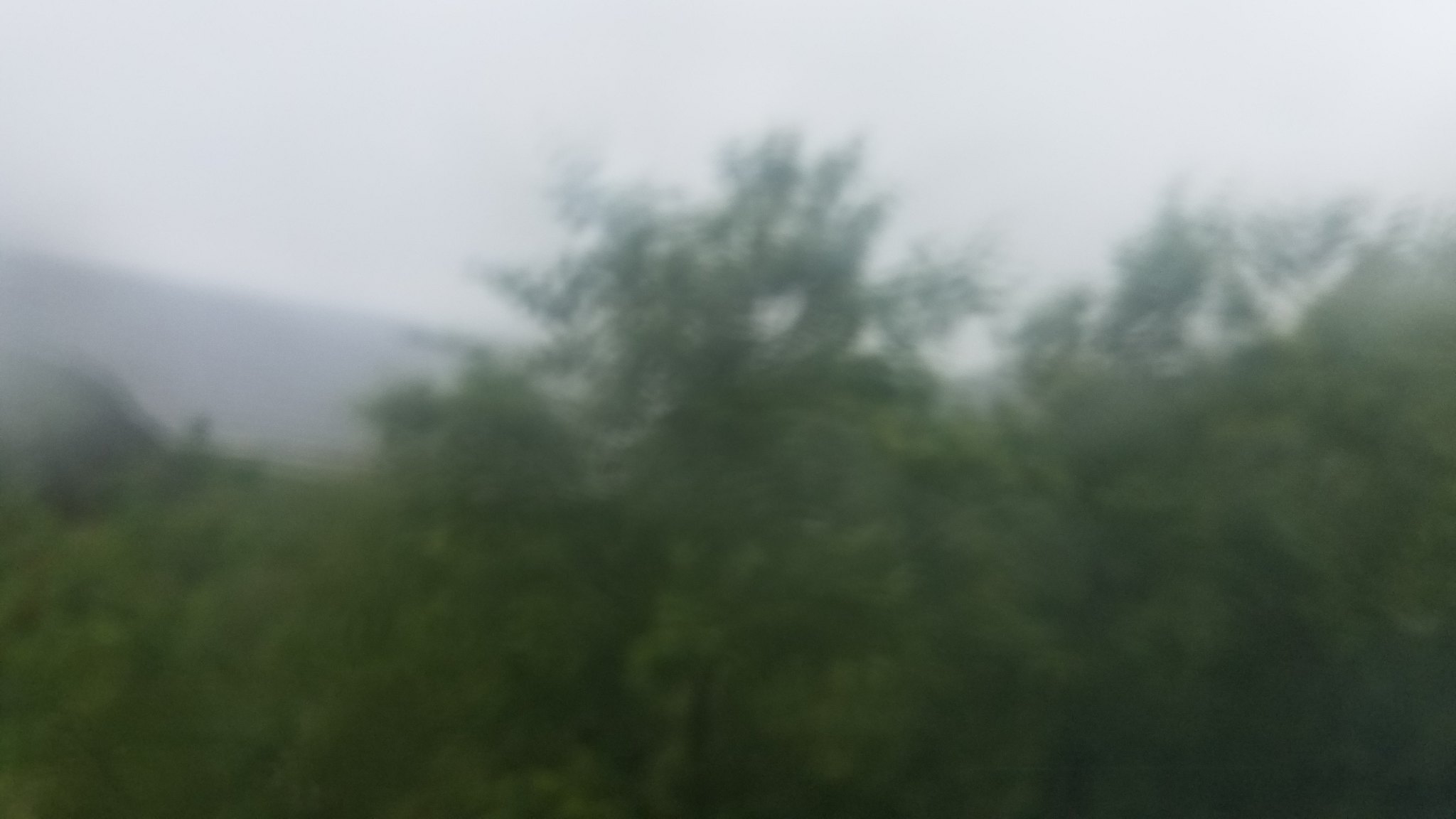A blurred image captures the hazy scene of a dense tree line, where lush green trees dominate the background. Despite the overall lack of clarity, one central tree stands out amidst the foliage, its myriad branches distinctly visible even through the blur. The canopy of this standout tree appears particularly full, contrasting with its obscured surroundings. Above the treetops, the sky peeks through, a serene backdrop to the verdant scenery. Toward the left side of the image, there is a vague, shadowy form that might be a distant mountain or another indistinct object. The overall effect is a dreamlike, cloudy portrayal of nature's serene beauty.